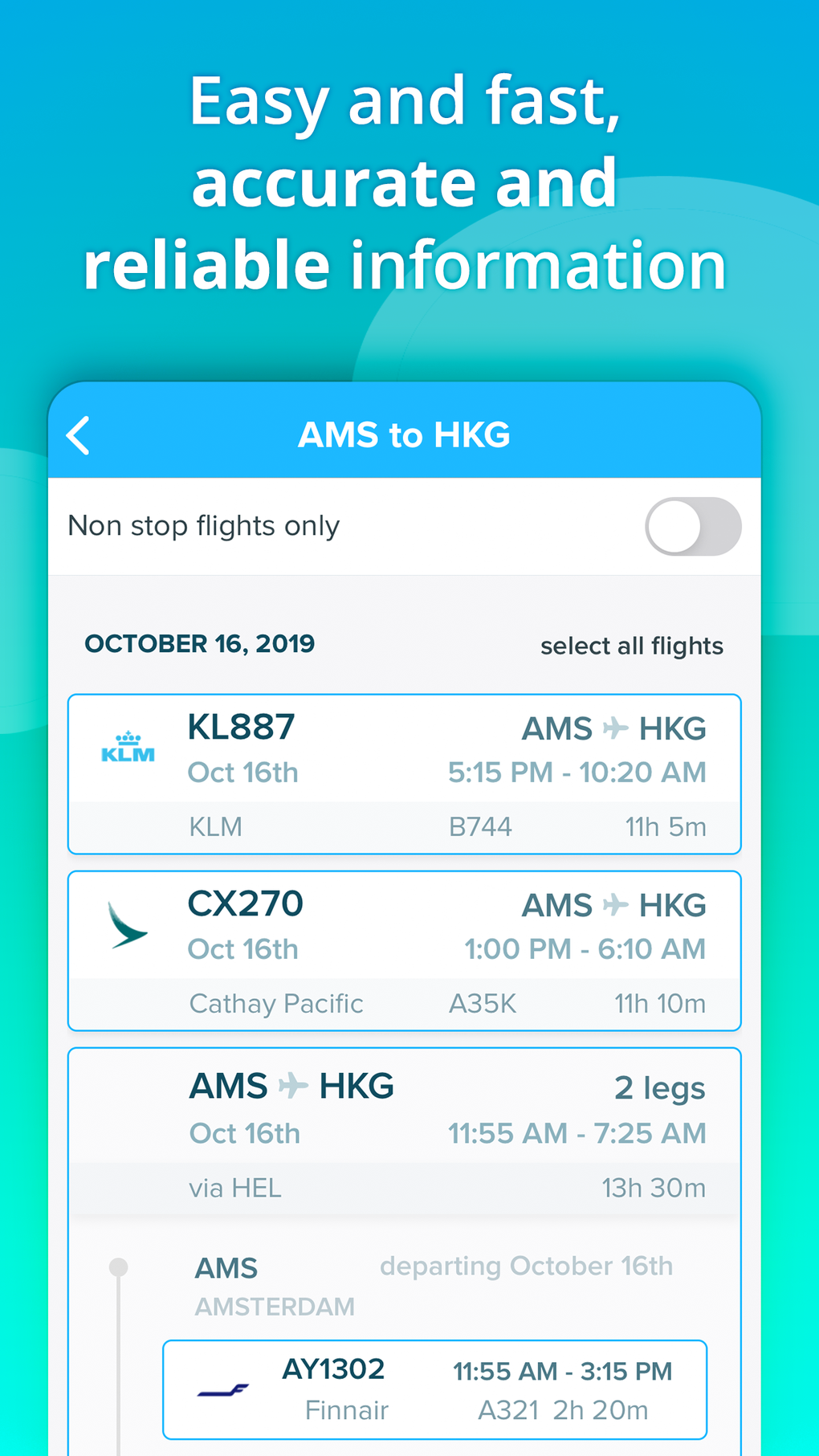The image features a blue background with a header at the top that reads "Easy and Fast Accurate and Reliable Information," with "Accurate and Reliable" emphasized in bold text. Below the header, an arrow points to the left with the text "AMS2HKG." Continuing downward, there is a section labeled "Non-stop Flight Only," which is currently deselected. The date "October 16, 2019" is noted along with the option to "Select All Flight."

Further down, flight details are listed:

- **KLM KL887:** From Amsterdam (AMS) to Hong Kong (HKG), departing at 5:15 p.m. and arriving at 10:20 a.m. on October 16, 2019. The flight is operated by a KLM Boeing 747-400 (B744) and has a duration of 11 hours and 5 minutes.
- **CX270:** From Cathay Pacific, departing on October 16, 2019, from AMS to HKG, operated by an Airbus A350-1000 (A35K). This flight departs at 1:00 p.m. and arrives at 6:00 a.m., with a duration of 11 hours and 10 minutes.